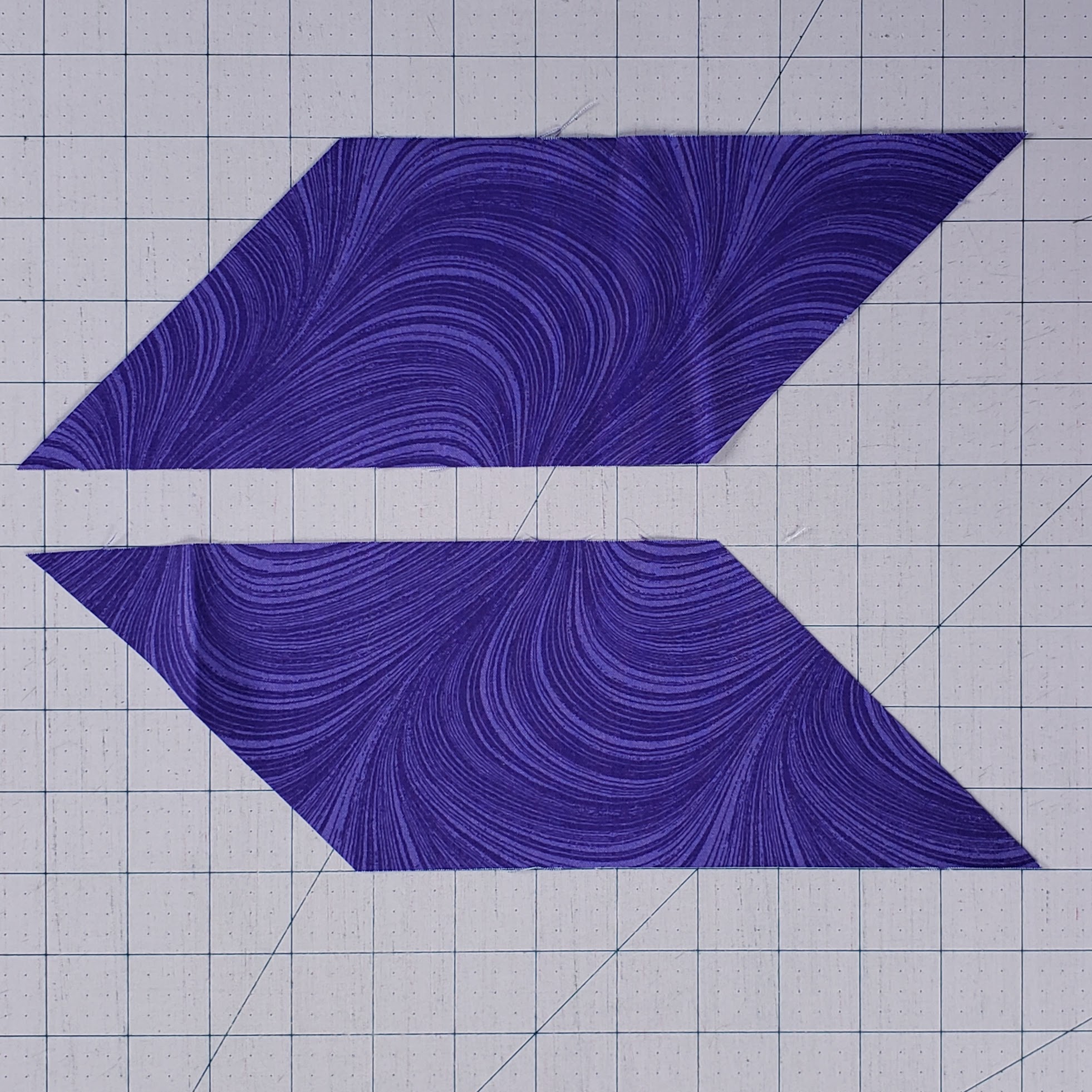This image features a top-down view of two purple fabric cutouts laid on a white and blue grid cutting board. The cutting board has a detailed grid pattern with lines and dots; each square in the grid contains nine blue dots and some angled blue lines cutting across from the bottom left to the upper right. The two pieces of fabric are both parallelograms that are mirror images of each other, with one at the top and the other at the bottom of the image, separated by a single row of grid squares. Each parallelogram has a swirling, curving pattern in various shades of purple, ranging from dark to lighter hues. The fabric exhibits some frayed threads along the edges, indicating its textile nature. The overall composition and mirrored placement of the fabric pieces make them resemble an arrow pointing to the left.